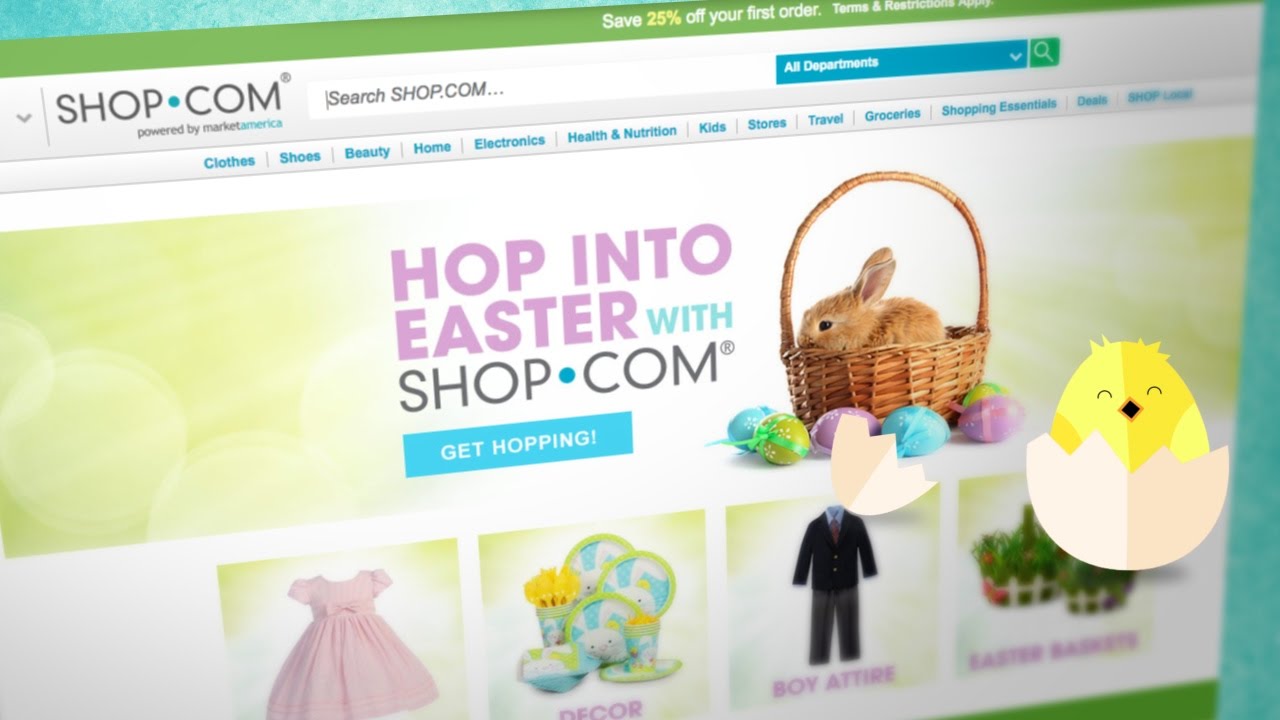The image depicts a slightly skewed screenshot of the shop.com website, with certain portions appearing blurred and edited with Photoshop overlays. At the top of the site, a prominent green menu bar displays a promotional message in white text stating, "Save 25% off your first order, terms and restrictions apply." 

Just below this, the official shop.com logo is positioned on the top left corner, adjacent to a white search bar outlined in gray text that prompts, "Search shop.com." To the right of the search bar, there's a blue dropdown menu labeled "All Departments," followed by a green magnifying glass icon signifying the search function.

Directly beneath this header, the navigation menu is presented in blue font, offering categories that include Clothes, Shoes, Beauty, Home, Electronics, Health & Nutrition, Kids, Stores, Travel, Grocery, Shopping Essentials, Deals, and another option partially blurred on the right side of the image.

The main body of the page features a festive image for Easter, showcasing a bunny in a woven basket. To the left of this image, text reads, "Hop into Easter with shop.com," accompanied by a blue button labeled "Get Hopping" inviting users to explore further.

Lower on the page, there are additional clickable buttons and images, though some content remains partially unreadable due to blurring. A pink dress is displayed with an illegible label beneath it, followed by bunny-themed plates under the category "Decor." Adjacent to this, a boy's suit and pants are labeled "Boy Attire," and nearby woven baskets are captioned "Easter something," though the text is indistinct. The image also includes a Photoshop overlay featuring a chicken and egg, which is prominently crafted over the existing visuals.

Overall, the screenshot offers a colorful and seasonally themed snapshot of the shopping website, albeit with some elements obscured and modified.